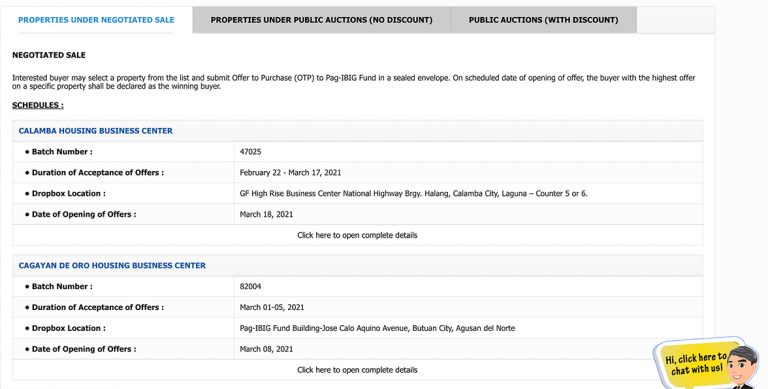Here is a cleaned up and detailed caption for the described image:

---

This is a screenshot of a webpage featuring a real estate portal with numerous details and user interaction elements. In the lower right corner, there is an animated drawing of a man's face, depicted as a white male with black hair, wearing a black suit of which only the top is visible. Adjacent to this illustration is a yellow box with the text, "Hi! Click here to chat with us."

The main content of the webpage is divided into various sections. At the top, three tabs are visible:
1. "Properties under Negotiated Sale" (currently selected)
2. "Properties under Public Auctions (No Discount)"
3. "Public Auctions with Discount"

Under the highlighted "Properties under Negotiated Sale" tab, a description is provided: "Negotiated Sale. Interested buyers may select a property from the list and submit an Offer to Purchase (OTP) to PAG-IBIG Fund in a sealed envelope on the scheduled date of opening of offers. The buyer with the highest offer on a specific property shall be declared as the winning buyer."

Following the description is a "Schedules" section, divided into two housing business centers:

1. **CALAMBA Housing Business Center**:
   - **Batch Number**: 47025
   - **Duration of Acceptance of Offers**: February 22 to March 17, 2021
   - **Drop Box Location**: GF High-Rise Business Center, National Highway, etc., Laguna Counter 5 or 6
   - **Date of Opening of Offers**: March 18, 2021
   - **Link**: "Click here to open complete details"

2. **CAGAYAN DE ORO Housing Business Center**:
   - **Batch Number**: 82004
   - **Duration of Acceptance of Offers**: March 1 to March 5, 2021
   - **Drop Box Location**: PAG-IBIG Fund Building, etc., Agusan del Norte
   - **Date of Opening of Offers**: March 8, 2021
   - **Link**: "Click here for complete details"

---

This new caption retains all the original information but presents it in a more organized and structured manner.